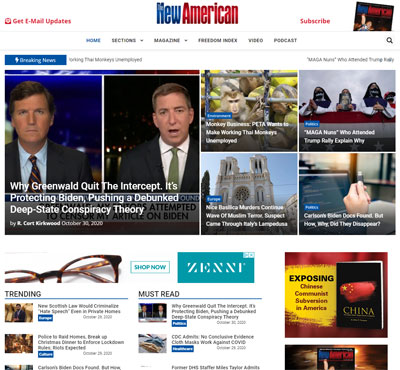The image showcases a webpage with a prominent headline at the top, "New American," displayed in blue and red colors. Below the title, there are two noticeable red buttons labeled "Get Email Updates" and "Subscribe." The webpage is divided into several sections: Home, Sections, Magazine, Freedom Index, Video, and Podcast. A blue "Breaking News" banner is also visible on the page.

The layout includes a variety of images and news headlines. The leading headline reads, "Why Greenwald Quit the Intercept? It's Protecting Biden, Pushing a Debunked Deep State Conspiracy Theory," authored by R. Kurt Kirkwood on October 30, 2020. Another headline highlighted is "Monkey Business, PETA Wants to Make Working Thai Monkeys Unemployed," accompanied by an image of monkeys.

Additionally, there are various advertisements scattered throughout the page; one ad prominently features a pair of brown eyeglasses. The webpage has a white background and visually distinctive images that correspond to their respective article headlines. The page also features sections for trending and must-read stories, providing a comprehensive array of current content to engage readers.